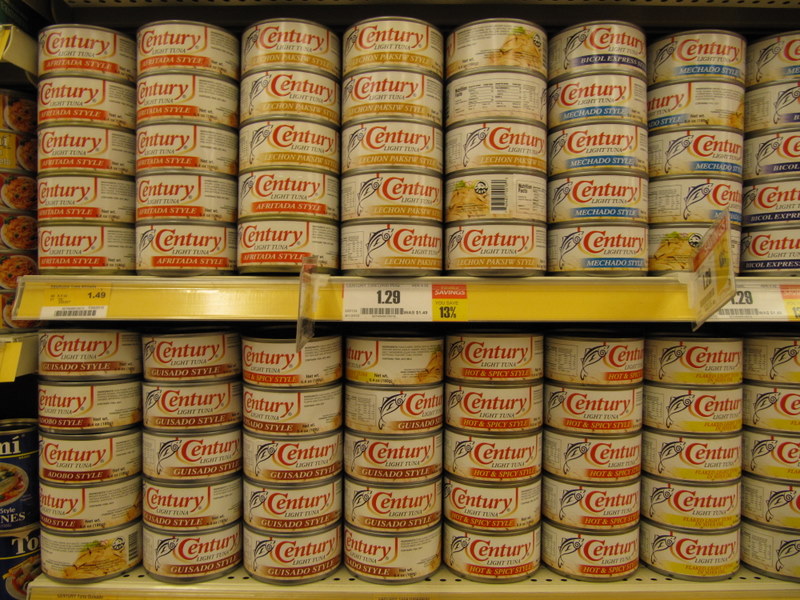The image depicts an assortment of tuna cans arranged on shelves. In the middle of the image, slightly towards the left, there was once a shell visible, marked by the term "sinus 1.49." Adjacent to this, in the center-right section, another marking reads "sinus 1.28," accompanied by a yellow rectangle indicating "13%." At the top of the image, multiple cans are displayed prominently. On the far leftmost tile, a red-labeled sentry can is visible, though the label’s exact wording is indistinct, with some yellow text present. To the far right, there appears to be a can labeled "meshado style," likely containing light tuna. The lower section of the image reveals a variety of cans with white labels, interspersed with cans bearing red and yellow labels.